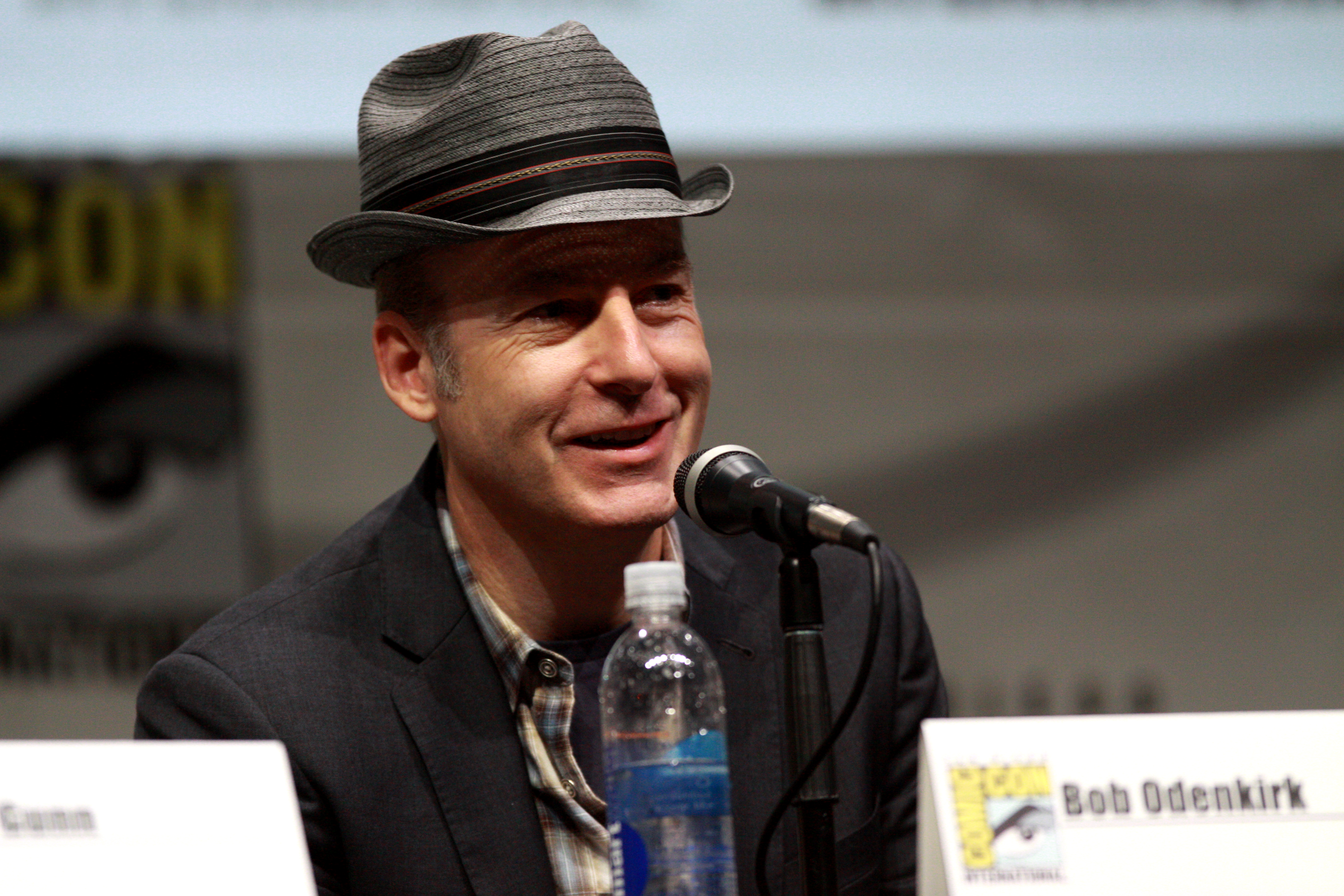The image features Bob Odenkirk, known for his roles in "Breaking Bad" and "Better Call Saul," seated at a panel, likely at a Comic Con conference. He is positioned behind a microphone and appears to be engaged, possibly talking or preparing a response, with a faint smile on his face. The actor, a middle-aged white male with gray hair, is wearing a distinctive gray hat adorned with a black band and some imprints at the top. His attire includes a black jacket over a flannel shirt, with a t-shirt underneath. A clear water bottle with a blue label is placed in front of him, alongside a triangular name tag that reads "Bob Odenkirk" in blue text. The background includes a Comic Con logo featuring an upside-down capital "L," a comic book drawing of an eye in the bottom right, and a projector screen above to the left.